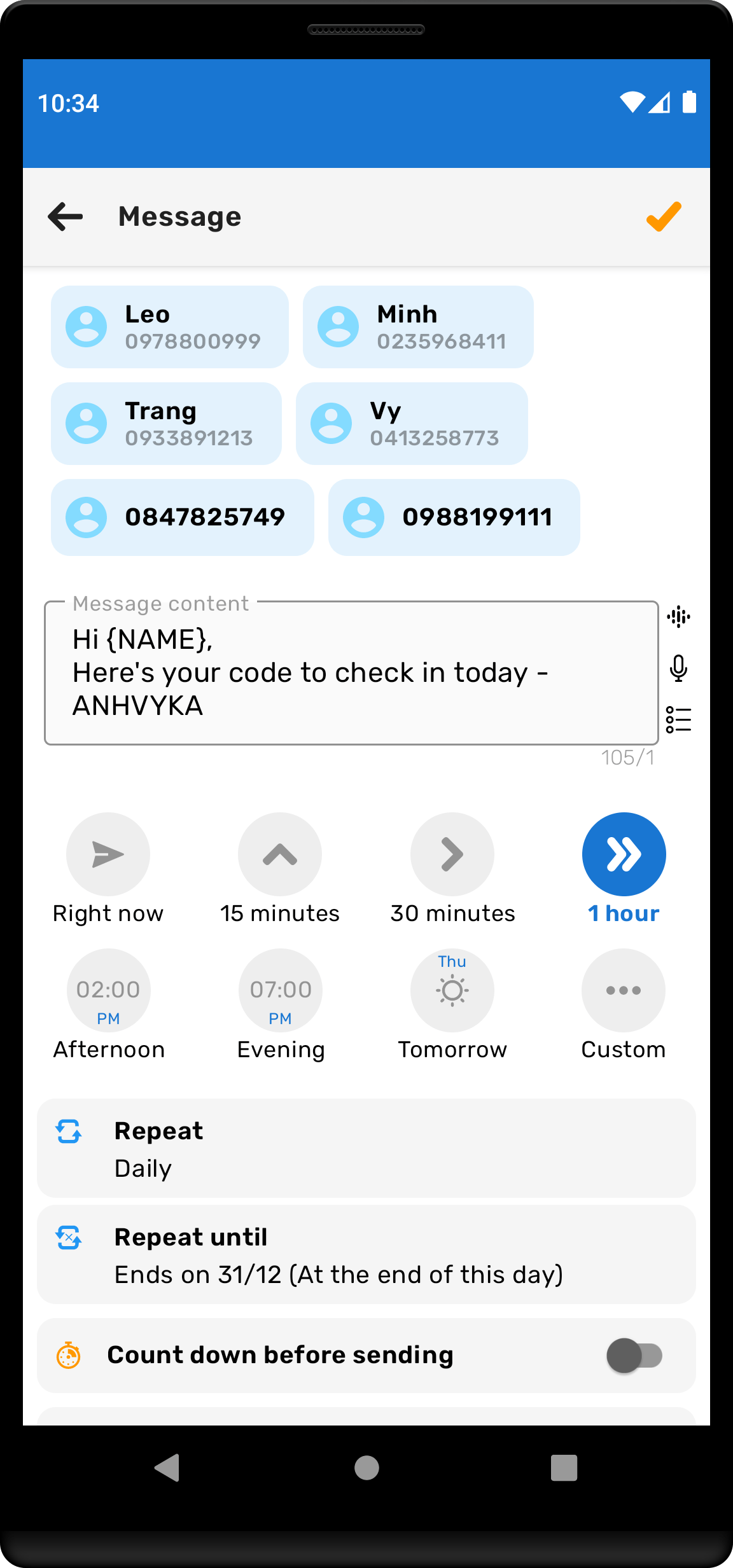In this image, a black, relatively square mobile phone displays an open app on its screen. At the top of the screen, there is a horizontal blue bar showing the time as 10:34. On the right-hand side of this bar, icons indicate cellular signal strength, Wi-Fi strength, and battery level.

Below this bar, there is a back arrow followed by the word "Messages" and an orange check mark. Underneath, there are six light blue pop-up boxes or cards arranged in two columns of three rows each, containing names and numbers. Each card includes a round person icon. 

In the first column, the top card reads "Leo," the middle card reads "Trang," and the bottom card only shows the number "0847825749." In the second column, the top card reads "Min," the middle card reads "Vi," and the bottom card only shows the number "0988199111."

Below these boxes, there is a text field labeled "Message Content," which contains the draft message, "Hi (Name), here's your code to check in today on Vika." Further down, various scheduling options for sending the message are shown: "Right now," "15 minutes," "20 minutes," "1 hour," "2 p.m. afternoon," "7 p.m. evening," "Thursday," "tomorrow," and "custom." Additionally, options for message repetition are listed: "Repeat daily" and "Repeat until ends on 31-12 at the end of this day." The final section includes a selection labeled "Count before sending."